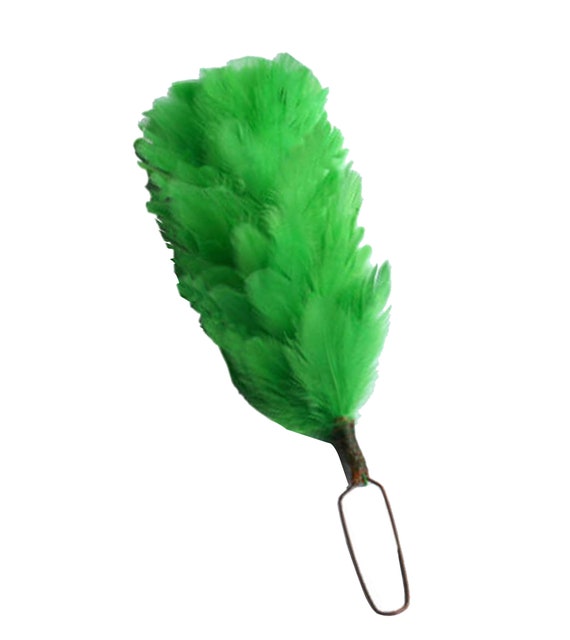The image depicts a handheld duster set against a pure white background. The duster features a black handle equipped with a black hook for easy hanging. Extending from the handle is a large wire ring that supports the main body of the duster, which consists of numerous green feathers. These feathers, predominantly a dark lime green, exhibit a gradient where lighter and whitish tones appear towards the top and deeper green shades are concentrated at the base near the handle. The feathers are arranged with their stems anchoring at the bottom and fanning out upwards. The object is oriented diagonally across the image, with the handle and hook positioned towards the bottom right and the feathered end extending to the top left corner, giving the duster a slightly elongated appearance.